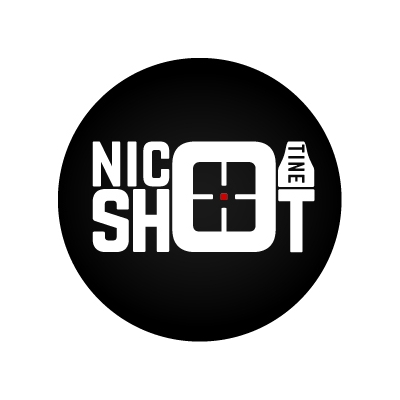In the image, we see a minimalistic logo set against a completely white background. At the center is a prominent black circle with distinctive white and red elements within it. The text "N-I-C" is positioned at the top left corner, followed by a large "S" and "H" beneath it. The letter "O" takes the form of a square that is as tall as the combined height of the letters on the left. Within this "O" is a bullseye target featuring four radial lines and a central red dot or square. To the top right of the black circle is a unique shape resembling a bottle or light bulb with the horizontal text "tined" in black. The bottom right shows the letter "T". Collectively, the elements spell out "Nic Shot," suggesting a scoped view, which possibly implies precision. The overall design appears to be a company logo, likely intended for use on a website or business card, reflecting the brand identity for a product named "Nicotine Shot."